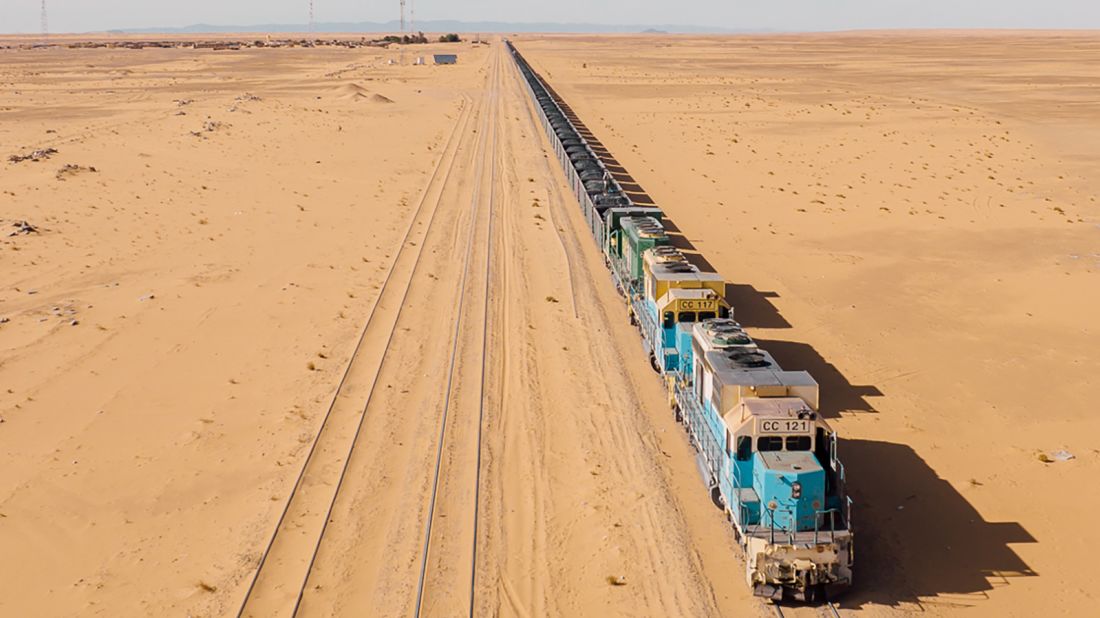The horizontally aligned rectangular image captures an expansive desert scene dominated by light brown, golden sand extending to a flat horizon. Three sets of railroad tracks slice through the barren landscape, running from the foreground to the background. On the right track, a lengthy train begins with a blue engine marked "CC121" with a gold top, located at the lower right corner. The train stretches into the distance, featuring a yellow car followed by a green one and many other open-top black cars, potentially filled with coal. The middle and left tracks are empty, enhancing the solitude of the vast, sandy expanse. A strip of cloudy gray sky is visible at the top, casting subtle shadows that emphasize the scene's daylight brightness. Some small landmasses appear faintly on the horizon, adding to the sense of isolation in this expansive, arid environment.